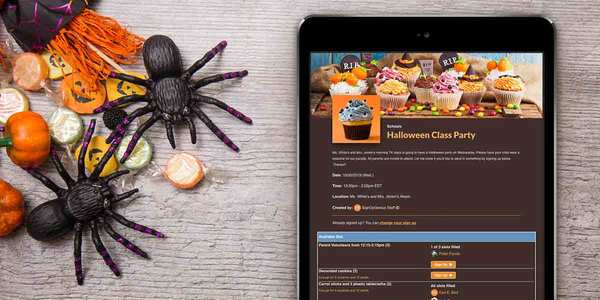The horizontal image features a smartphone placed on a grayish-brown wooden table or bench, adorned with intricate wood grains and lines. The surface is decorated with Halloween-themed items, including small spiders, pumpkins with faces, decorative gourds, and assorted candies, all clustered in the left-hand corner of the frame. Positioned to the right of these festive decorations, a black smartphone occupies the right-hand side of the image, with its display partially visible. The phone's screen shows a digital flyer for a Halloween class party, featuring a layered image of Halloween-themed cupcakes. The flyer includes the bold heading "Halloween Class Party," followed by slightly blurry white text detailing the event. Towards the bottom, a blue rectangular button and additional white and orange text provide further interactive options and information about the celebration.